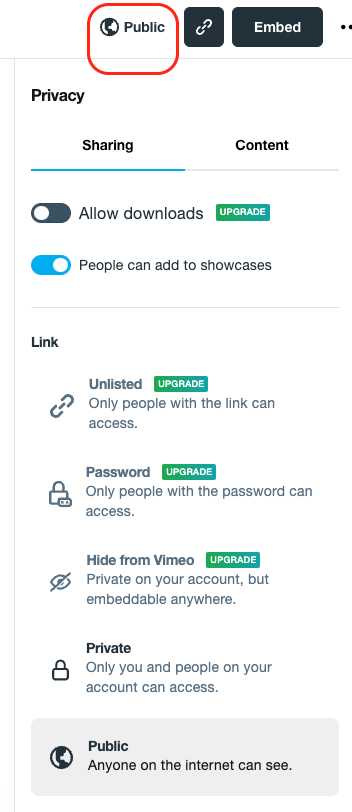The image showcases interface options on what appears to be a video-sharing platform, most likely Vimeo, given the context and design elements described.

At the very top of the interface on a white background, there's a globe icon signifying public visibility, accompanied by the word "public" encased in a red box. Below this, the word "privacy" is displayed in black font. 

Following "privacy," there are several underlined and colored elements indicating different options: "sharing" is underlined in blue, and "content" is underlined in gray.

Beneath these options, there's a section labeled "allow downloads" with an associated toggle switch. This switch consists of a small white circle within a black bubble, positioned to the left, indicating that the download option is currently turned off. Adjacent to this, there's a small green rectangle with the word "upgrade," likely indicating that toggling this option requires a premium account.

Further down, the image indicates permissions for adding to showcases. This section has a blue toggle, with the white circle slid to the right, suggesting that this option is currently enabled.

A horizontal gray line divides the next section, which starts with the word "link" in black letters. This section contains the option "unlisted," also tied to an upgrade feature highlighted in a green box. Text clarifies that only people with the link can access the video.

Following this, there's a "password" option requiring an upgrade, again marked by a green rectangle. Only individuals with the password can access the video when this setting is enabled.

Next is the "hide from Vimeo" option, also tied to an upgrade and denoted by a green rectangle, indicating that the video will be private on the user's account but embeddable elsewhere.

Beneath this, there's a "private" setting represented by a lock icon, ensuring that only the user and people on their account can access the video.

At the very bottom, the interface displays a gray square with a globe icon and the word "public," indicating that the video visibility setting is currently enabled for anyone on the internet.